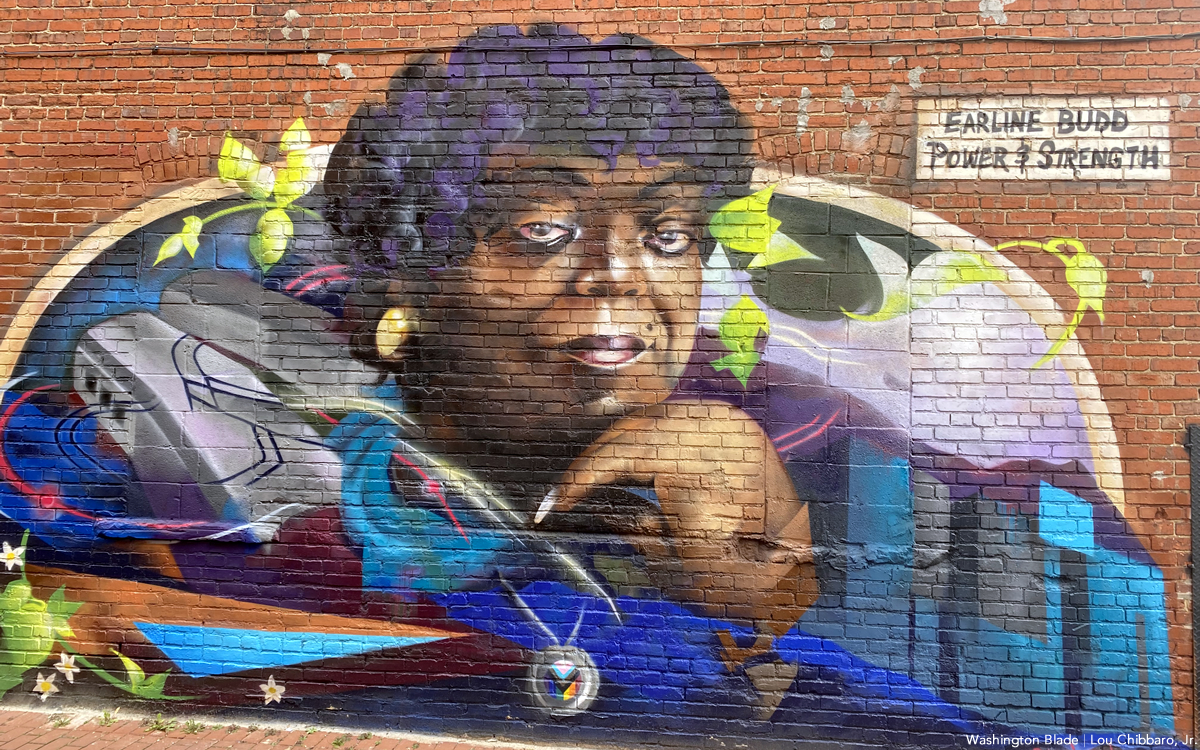This vibrant and detailed mural, painted on the side of an old light brownish-red brick building, depicts a strong and dignified African American woman named Earline Budd. Her image is framed by a white arch, with her curly black and purple hair spilling over the top. Her facial features are strikingly detailed, from her expressive eyebrows and eyes to her dark brown lips. She is holding her chin with her left hand, which rests elegantly beneath her face.

Earline Budd is adorned with a solid gold oval-shaped earring on the right side of her face, and she is dressed in a blue collar that wraps around her neckline. A silver necklace featuring multicolored gems, predominantly blue, yellow, and purple, lies across her chest. 

To further highlight her presence, the background includes green vine-like plants and musical notes that add an element of texture and rhythm to the scene. Below these elements, a mix of what appear to be buildings with roofs, windows, and pillars blends into the mural's aesthetic, creating a layered urban backdrop. 

Floral designs and green plants rise from the bottom left, adding a touch of nature. A pathway that resembles a brick sidewalk stretches along the lower edge, while some surrounding structures, including a structure with red arches and another that appears to be a vehicle, enrich the scene with a sense of community and daily life.

In the upper right corner of the mural, the text boldly declares "Earline Budd," followed by the words "Power and Strength," encapsulating the mural's tribute message. Additional subtle details, such as light posts and what could be transit vehicles, merge seamlessly into the complex yet beautiful cityscape, emphasizing the dynamic environment in which Earline Budd's legacy of resilience and empowerment is celebrated.